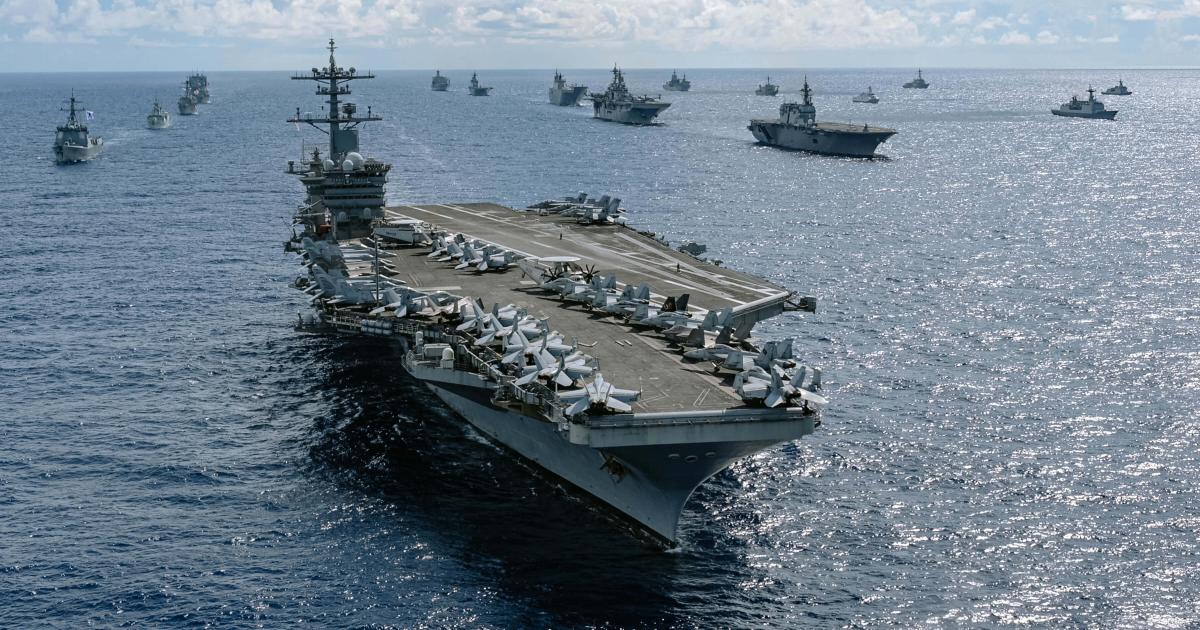An overhead shot captures a vast military fleet navigating through the dark blue ocean, leaving distinctive trails in the water behind them. Dominating the foreground is a colossal gray aircraft carrier, featuring multiple decks, prominent antennas, and an array of fighter jets strategically positioned on its deck. The fleet consists of various other military ships, including gunboats, which follow the aircraft carrier in a coordinated formation. The surrounding waters appear calm, reflecting the bright sunlight that filters through scattered clouds in the blue sky above. Although some ships seem to be approaching, others are departing, creating a dynamic and expansive scene in the open sea.